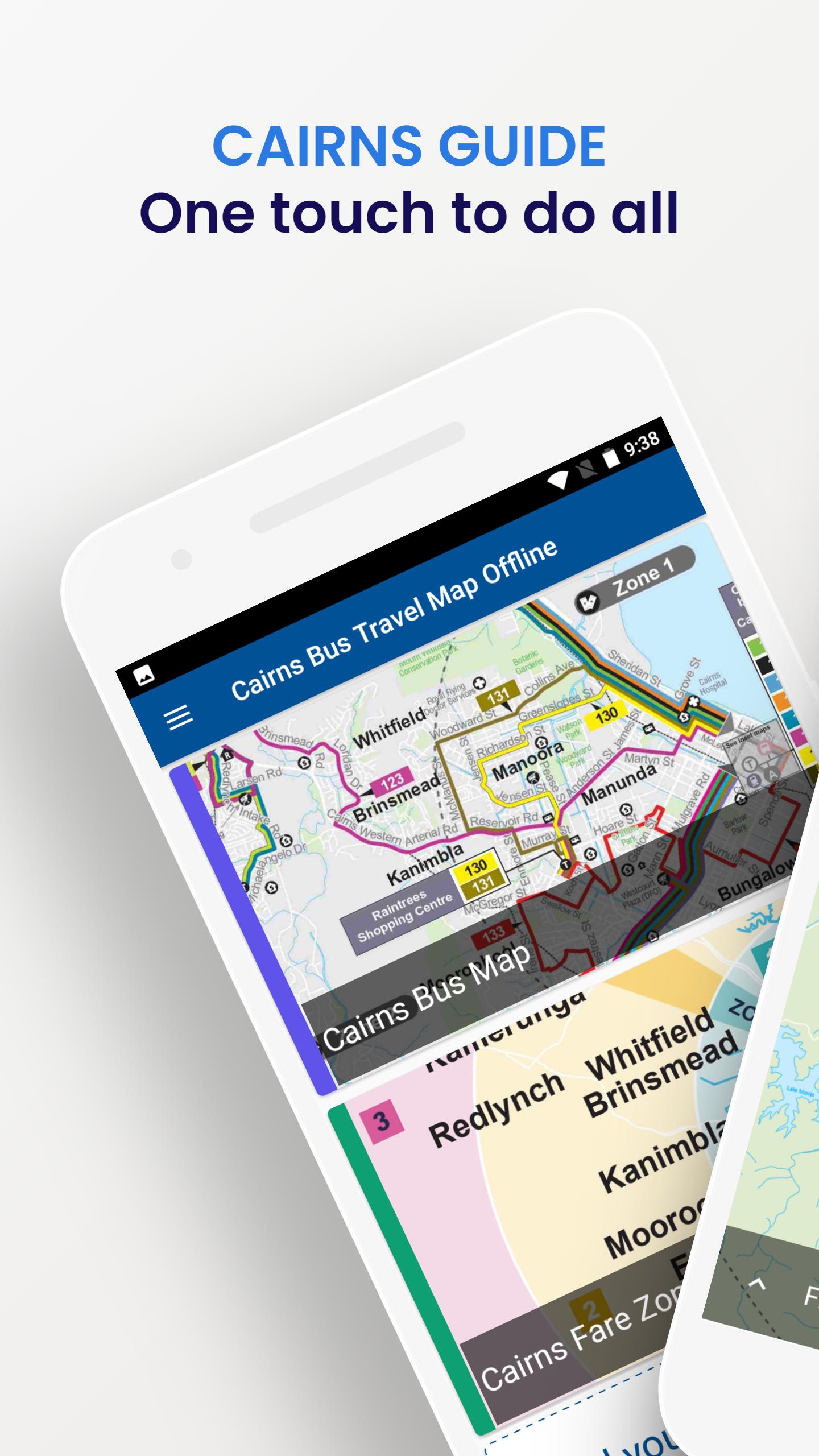The image features a predominantly white background, which has a folded appearance at the bottom right corner, resembling a piece of paper. At the top, bold blue text reads "CAIRNS guide," likely indicating "Cairns Guide." Beneath this, in black text, it states, "One touch to do all."

Central to the image is a depiction of a white cell phone with a long black bar at the top, displaying a white battery icon. Below the battery, on a blue line, the words "Karen's Bus Travel Map Offline" are displayed, accompanied by three tiny horizontal white lines to the left, suggesting a menu icon.

The screen of the phone showcases a map with numerous pink lines crisscrossing the area, displaying notable names such as Whitfield, Brinsmead, Menuda, and Cambia. Within a gray circle, the text "Zone 1" is visible, signifying a specific fare zone. 

Underneath the map, more text reads "Karen's Bus Map," overlaying a background adorned with pink and yellow hues and a green line along the side. Several towns are listed, including Red Lynch, Whitfield, and Brinsmead.

At the very bottom of the image, within a gray rectangle, the text "Karen's Fare Zone" is displayed, likely indicating the designated fare zones for the bus map service.